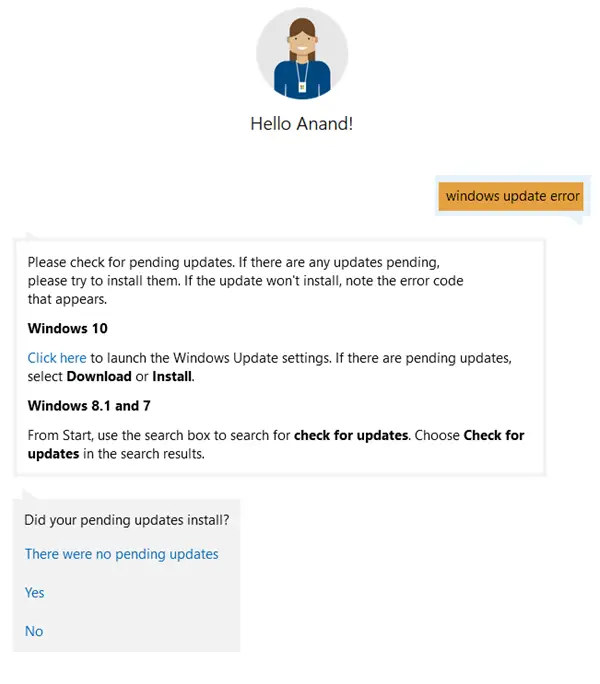In this screenshot, we observe an interactive chat interface, likely with a chatbot. At the top of the screen, there is a profile icon—a light gray circle featuring an illustration of a woman with brown hair, wearing a blue shirt and a lanyard, possibly displaying a badge. Below the icon, the text "Hello, a nod" appears in standard black font.

The interface primarily uses black font, with certain instructions and links highlighted in blue. The background of the interface is entirely white. To the right of the introductory phrase, "Hello, a nod," we find an orange button labeled "Windows Update Error."

In the lower left section below this button, there is a detailed instruction box. It advises users to "Please check for pending updates. If there are any updates pending, please try to install them. If the update won't install, note the error code that appears." Below this information, "Windows 10" is prominently displayed in bold black font, followed by a blue hyperlink that says "Click here to launch the Windows Update settings." Instructions continue, stating that if there are pending updates, users should select "Download" or "Install," with both terms emphasized in bold.

Further down, we see another section titled "Windows 8.1 and 7" in bold black font. The instructions here guide users to, "From Start, use the search box to search for 'check for updates.' Choose 'check for updates' in the search results," with "check for updates" highlighted in bold.

At the bottom of the interface, there is a light gray box asking, "Did your pending updates install?" Three response options are provided: "There were no pending updates," "Yes," and "No."